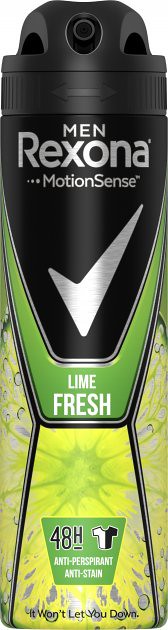This is an image of a men's antiperspirant deodorant spray can from the Rexona MotionSense line. The can features a sleek black lid with a spray nozzle on top. The upper section of the can is predominantly black, adorned with a silver checkmark that is outlined in green. Just below the checkmark, the label reads "Lime Fresh." Also prominently displayed is a green mark indicating "48H" for 48-hour protection. Below this, there is an illustration of a t-shirt, split into half white and half black, signifying the product's antiperspirant and anti-stain properties. Beneath the t-shirt icon, the words "Antiperspirant Antistain" are printed. At the bottom of the can, the slogan "It won't let you down" is clearly visible. The design also includes a vibrant tie-dye burst of yellow in the central area, along with small water droplets scattered along the sides of the can, adding a visually appealing touch.